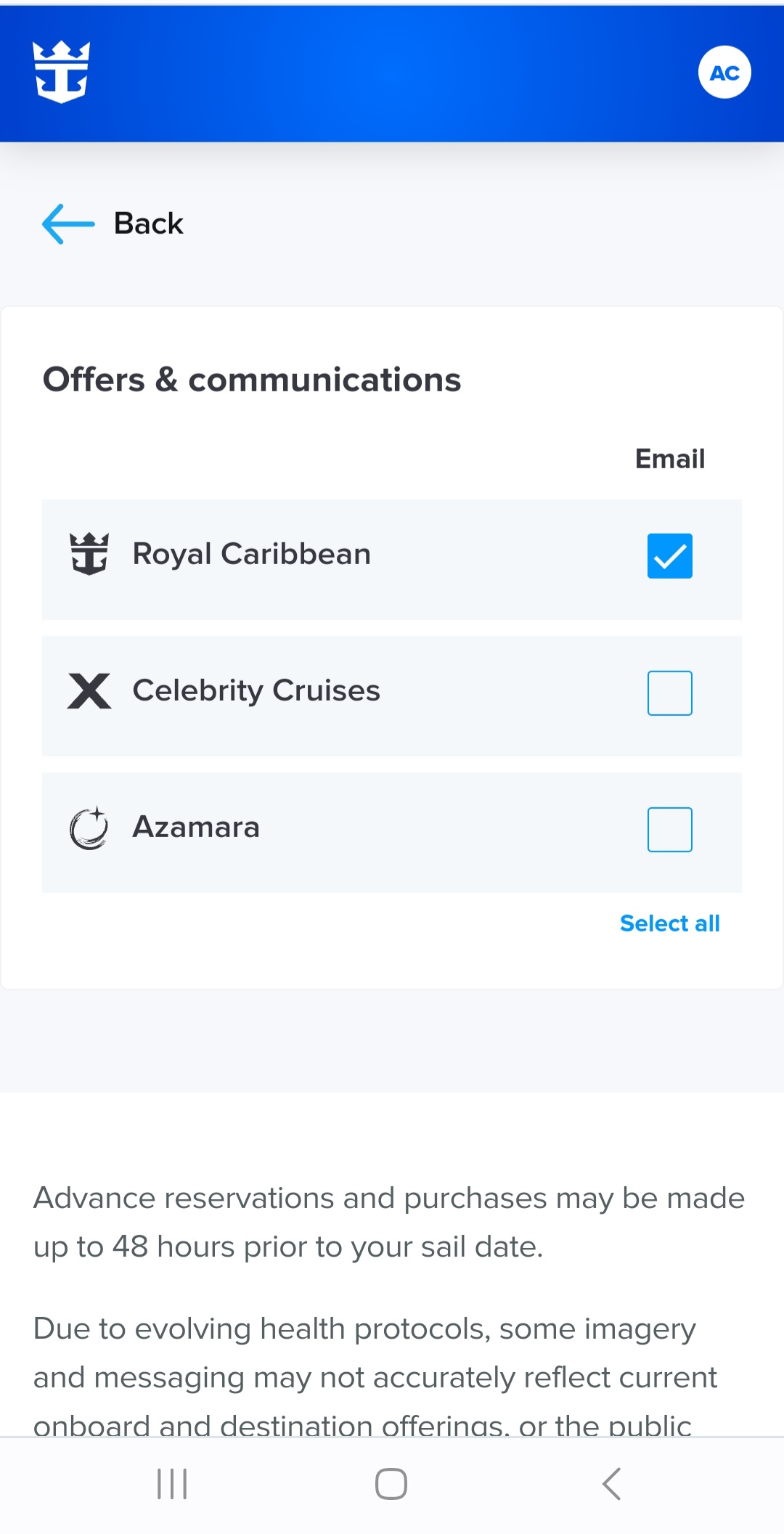**Detailed Caption:**

This is a screenshot from a cell phone displaying a particular section of an app or mobile web page, identifiable by a distinct blue header along the top. On the left side of the header, an icon featuring a white anchor topped with a crown is prominently displayed. To the right of this icon is a white circle containing the letters “AC”.

Beneath the blue header, a gray strip features a left-pointing blue arrow accompanied by the word "Back". Following this is a white section labeled "Offers and communications". The main body of this area is divided into three light blue horizontal bars.

The first bar is labeled "Royal Caribbean" and carries the same anchor and crown icon. On its right side, it has the word "Email", followed by a blue checkbox marked with a white tick. Below this, there is an "X" to deselect.

The second bar is labeled "Celebrity Cruises"; its box next to "Email" is currently unchecked. Similarly, the third bar marked "Azamara" has an unchecked box as well.

An option to "Select All" appears below these three selections. 

At the bottom of this section, in smaller print, it states: "Advanced reservations and purchases may be made up to 42 hours prior to your sail date. Due to evolving health protocols, some imagery and messaging may not accurately reflect current onboard and destination offerings...". The text truncates here.

The bottom navigation bar of the phone screen displays three common icons: three horizontal lines (likely to indicate a menu), a square, and an arrow.